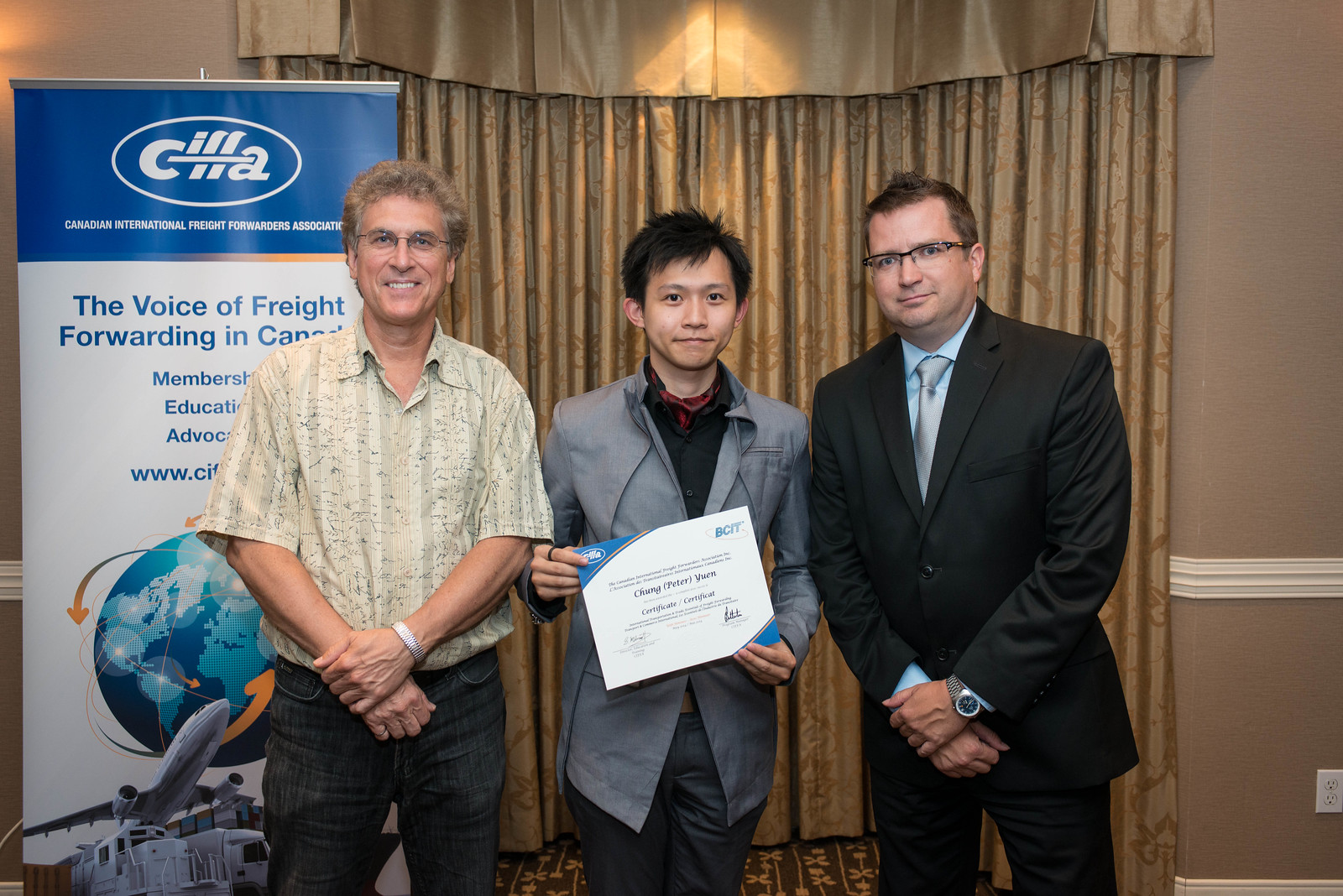This photograph captures an award ceremony featuring three men standing indoors. Central to the image is Chung "Peter" Yuen, who is being presented with a certificate from BCIT. Peter, an Asian man with short black hair, is holding the certificate, which features blue accents in the upper left and bottom right corners. He is dressed in a gray (almost silver) coat and black pants.

To the left of Peter, a Caucasian man wearing glasses and a short-sleeved cream-colored shirt with a design, along with black jeans, is smiling. Behind him, a poster for the Canadian International Freight Forwarders Association is prominently displayed, showing a globe and vehicles, and text advertising "the Voice of Freight Forwarding in Canada." The poster is set against brown curtains with a design.

On Peter's right, another Caucasian man is dressed in a black suit, paired with a blue shirt and a blue tie. He is also wearing glasses and a watch. The warm setting with brown curtains in the background adds a formal yet cordial atmosphere to the occasion.